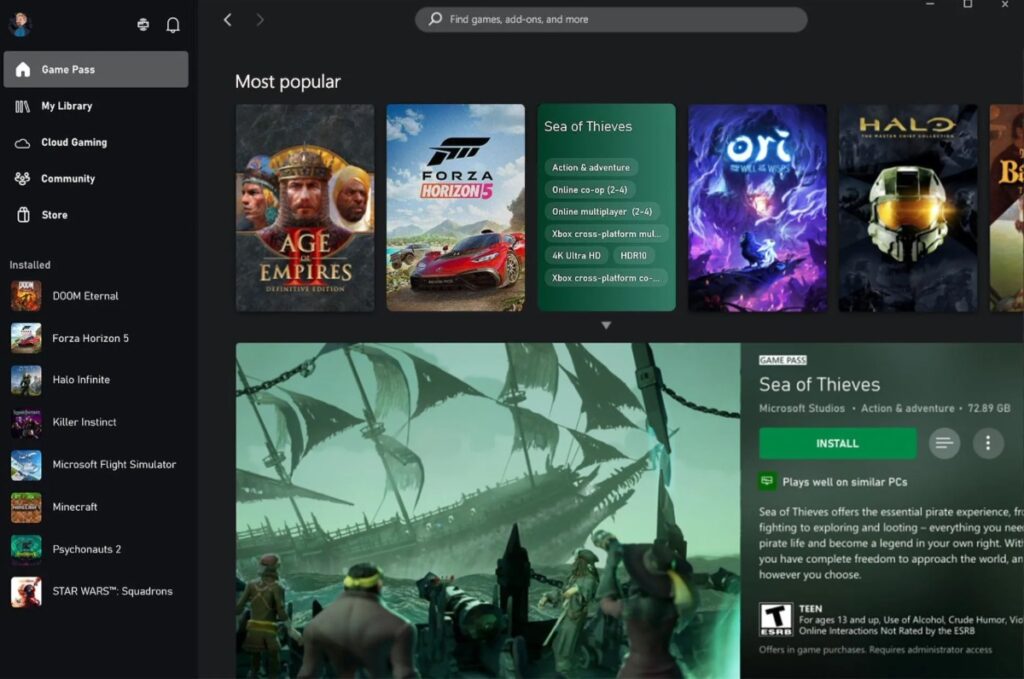The image is a detailed screenshot from a video game app or website interface. In the top left corner, an icon representing a person likely indicates the account menu. Beneath this, there's a vertical column featuring several icons: a house labeled "Game Pass," a bookshelf labeled "My Library," a cloud labeled "Cloud Gaming," an icon of three people for "Community," and a shopping bag for the "Store."

Further below, a list of installed games is displayed, including Doom Eternal, Forza Horizon 5, Halo Infinite, Killer Instinct, Microsoft Flight Simulator, Minecraft, Psychonauts 2, and Star Wars Squadrons.

On the right side, occupying the majority of the screen, a search bar sits at the top. Below it, a row of the most popular games is showcased, featuring Age of Empires 2, Forza Horizon 5, Sea of Thieves, Ori, and Halo. Sea of Thieves is currently selected, revealing detailed information below: it’s part of Game Pass, categorized as an action-adventure game from Microsoft Studios, with a size of 72.89 gigabytes. Additionally, there's a green install button along with a brief description of the game.